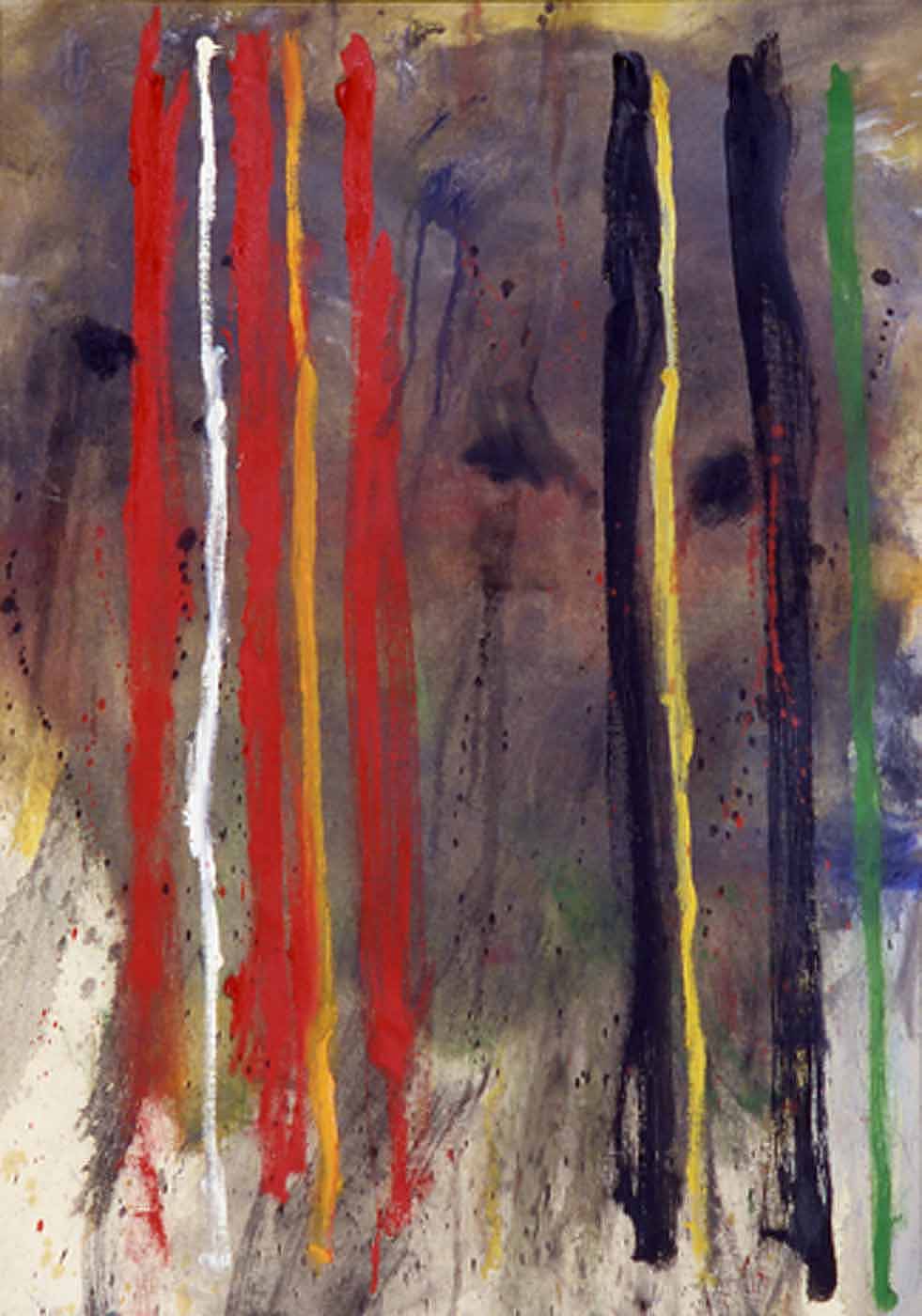The image is a highly abstract modern painting dominated by vertical ribbons and splattered patterns of various colors. The background features muted shades of gray and hints of purple and yellow, giving it a textured, almost expressionistic quality. There are two main sets of ribbons; in the left set, alternating thick red lines are interspersed with thinner white and yellow stripes. In the right set, vibrant blue lines flank thinner yellow and green stripes, with occasional splotches of red, blue, and other colors breaking the continuity. The arrangement suggests movement, resembling brush strokes and paint splatters that create a dynamic and somewhat chaotic appearance. Overall, the painting lacks concrete objects, focusing instead on the interplay of colors and textures, giving it the feel of a spontaneous, youthful artwork.